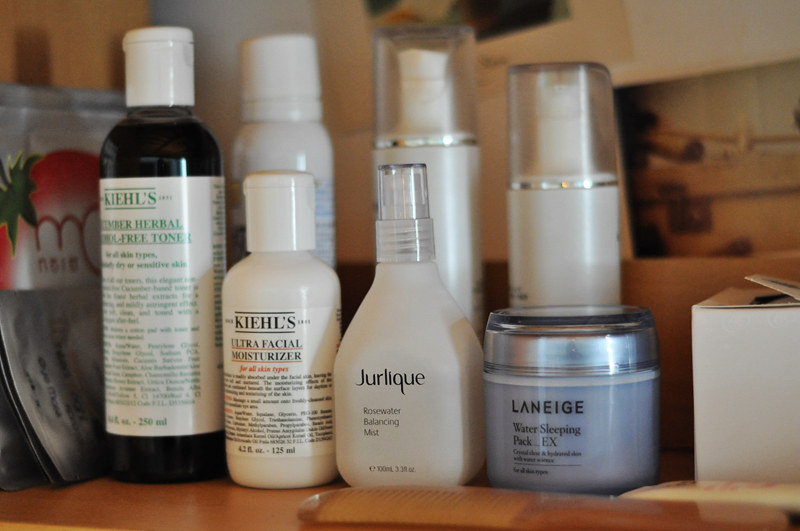The image features a collection of beauty products, predominantly marketed to women, displayed on a counter. Prominently visible are seven products, though only four are legible: Kiehl's Herbal Extract Alcohol-Free Toner and Kiehl's Ultra Facial Moisturizer, Jolique Rosewater Balancing Mist, and Laneige Water Sleeping Pack. The products are nestled closely together, with additional spray bottles partially obscured in the background. The backdrop includes an out-of-focus wall with indistinct items and a partially visible white box to the right, adding to the bathroom or vanity setting's ambiance. The labels on some products are in French, suggesting a touch of international or high-end allure.